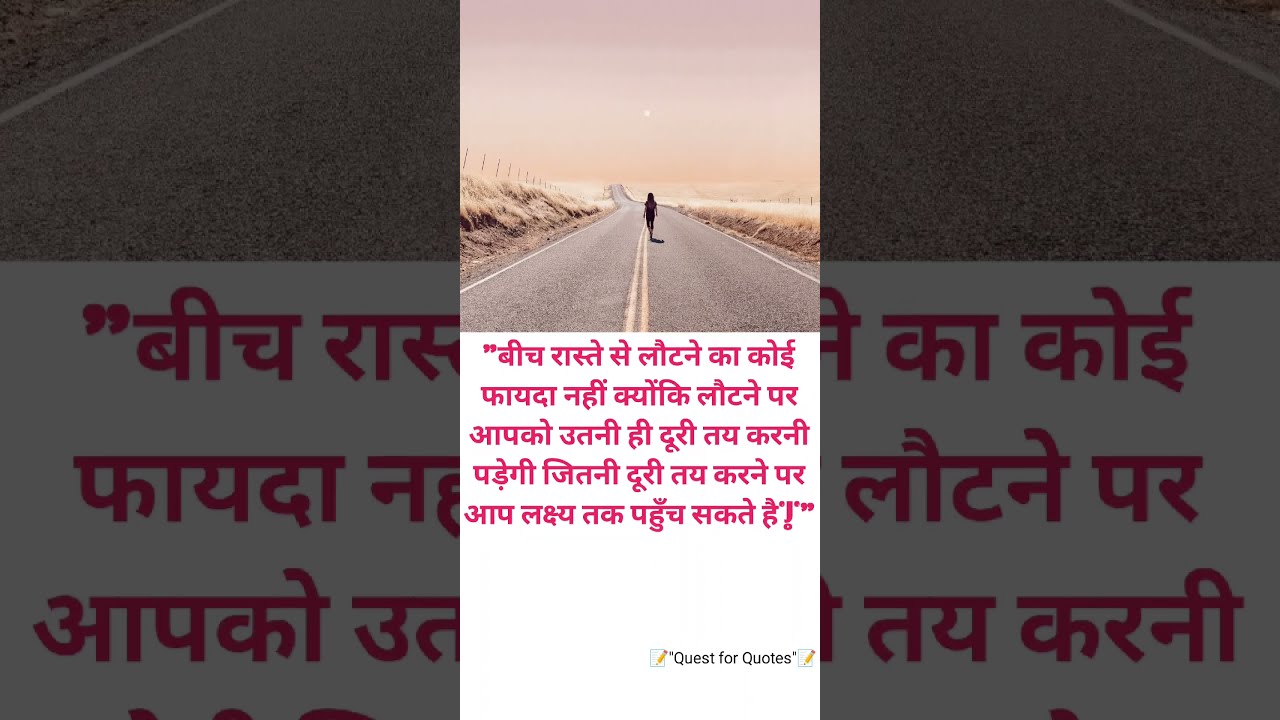The image, which appears to be a still shot from a video, depicts a desolate two-lane blacktop highway stretching straight into the horizon, bordered by dull brown vegetation resembling dried prairie grass. The scene is backlit with a hazy sky displaying shades of brown, orange, and pink, suggesting a dusty atmosphere. In the foreground, a woman is seen from behind as she walks down the center of the road, casting a shadow behind her onto the pavement. The highway is distinguished by double yellow lines in the middle and white lines on the sides. To the left and right, there are gradual embankments topped with fences. On the left side, the embankment has dried green grass, while the right side's incline is less steep. The sky features what might be a small, obscured sun in the distant horizon. Below the main image, there is a section with Asian script in red and the text "quest for quotes" at the very bottom. The entire composition is framed within a larger rectangle, where the borders are magnified and slightly grayed-out elements of the main image, creating a cohesive border effect.